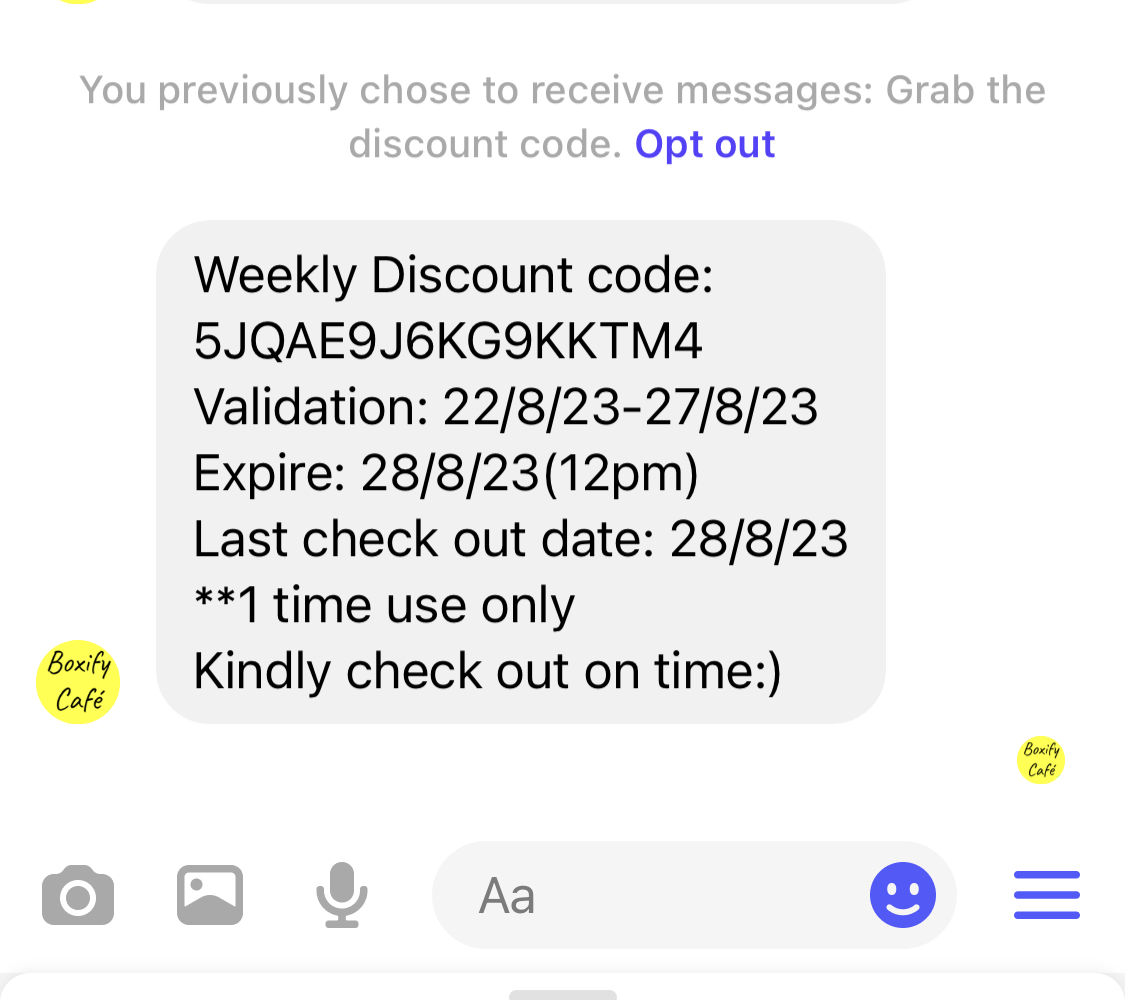The image depicts a screen capture of a messaging app interface on a white background. The main content of the message reads, "You previously chose to receive messages. Grab the discount code," followed by a blue-text option to "opt out." Below this, there is a gray box containing a weekly discount code presented as a string of letters and numbers. Important details within the gray box include the validation period "22-8-23 to 27-8-23" and the expiration date and time "28-8-23 at 12 PM." Additionally, it mentions that the code is for one-time use only, indicated by two asterisks, and advises users to check out on time, ending with a text-based smiley face ":)".

The message appears to be sent from 'Boxify Cafe,' indicated by a yellow circular logo with the text "Boxify Cafe" on the left side of the message and the same logo at the bottom right. The bottom interface of the messaging app shows icons for a camera, a photo, a microphone, a text input box with formatting options, an emoji button, and a hamburger menu button on the far right.